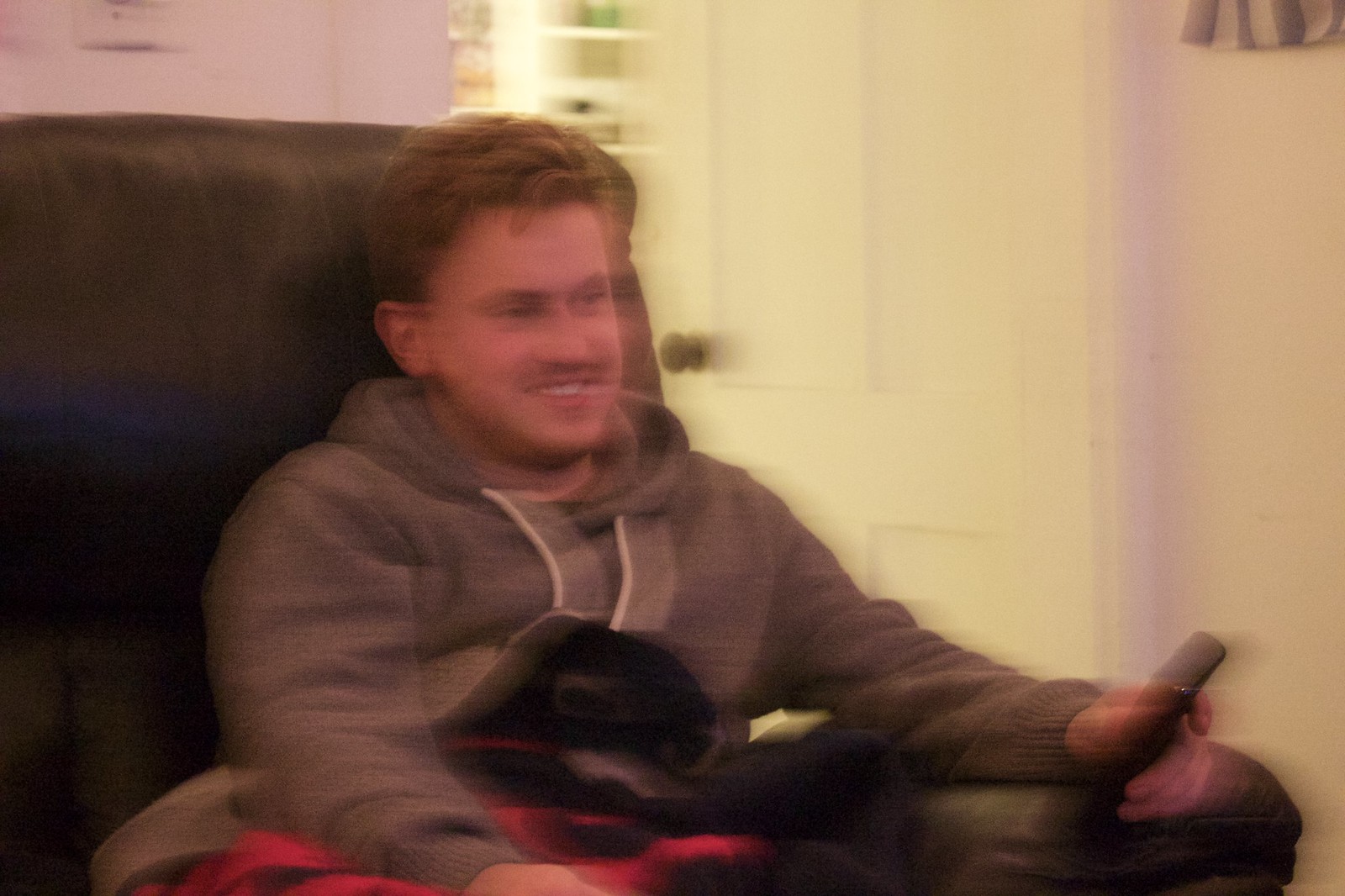In this blurry and distorted photograph, a young man, likely between 20-25 years old, is captured sitting in a leather recliner or couch, wearing a gray hooded sweatshirt with white laces. He has short, brownish-red hair and a faint five o'clock shadow, and he is smiling as he looks off to the right. His left hand holds a black object, possibly a TV remote or cell phone, while his right arm is draped over a small black dog that also has a red blanket resting on it. The background reveals white walls, a white door behind him, and a light source positioned above his head. Despite the low quality and out-of-focus nature of the image, the man's happy expression while watching TV with his pet is clearly evident.